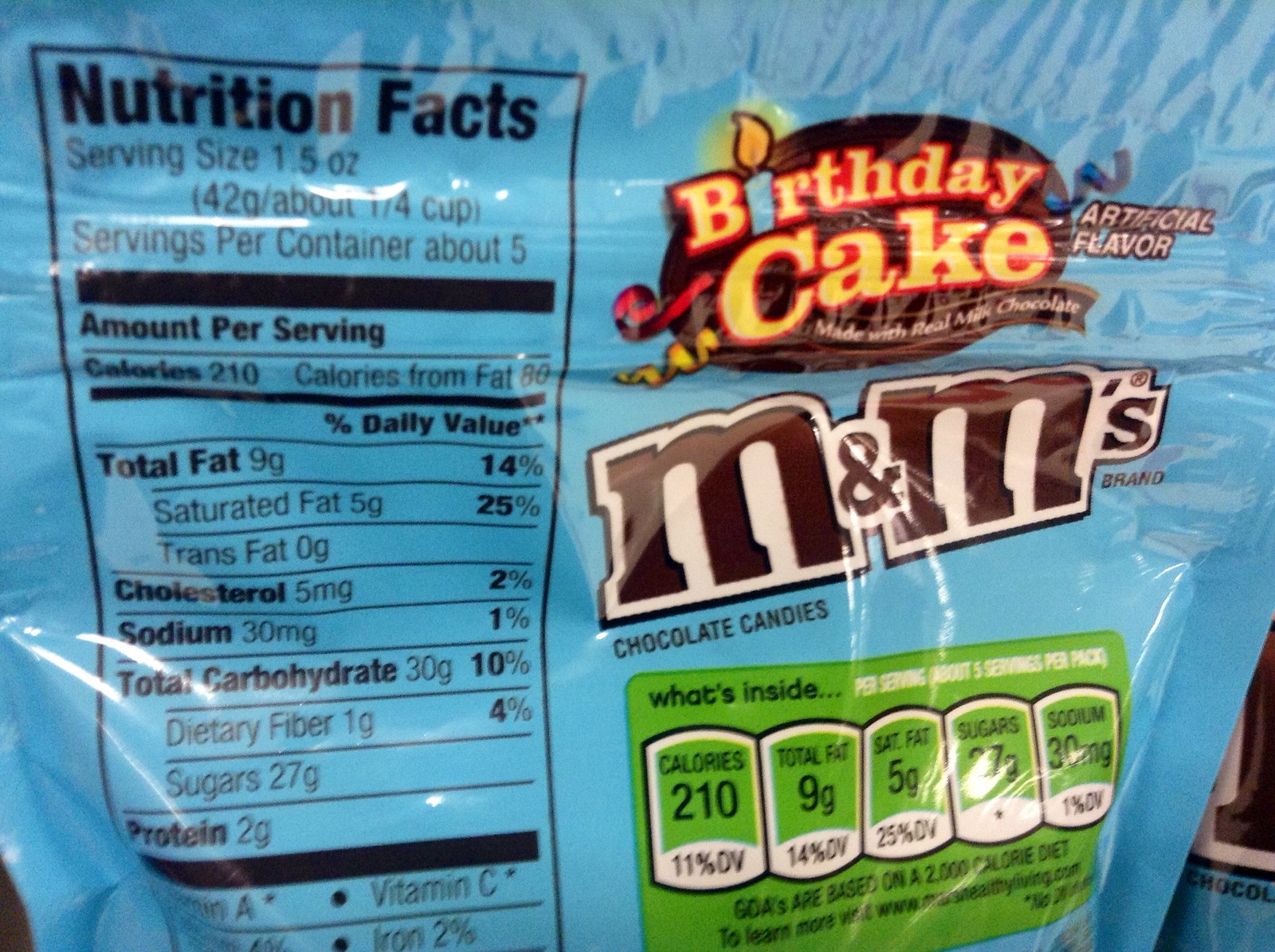The image features the back of a larger, Carolina blue bag of Birthday Cake M&M's, indicating it contains five servings. The traditional brown M&M's character is displayed on a white background. Prominently visible is a green shortcut nutritional label with black and white lettering, summarizing key information such as calories, total fat, saturated fat, sugars, and sodium per serving. The detailed nutrition facts box includes black markings and follows conventional labeling norms. The bag appears to be resealable based on its shape, suggesting it's designed for multiple uses despite containing a total of over 1,000 calories (210 calories per serving).